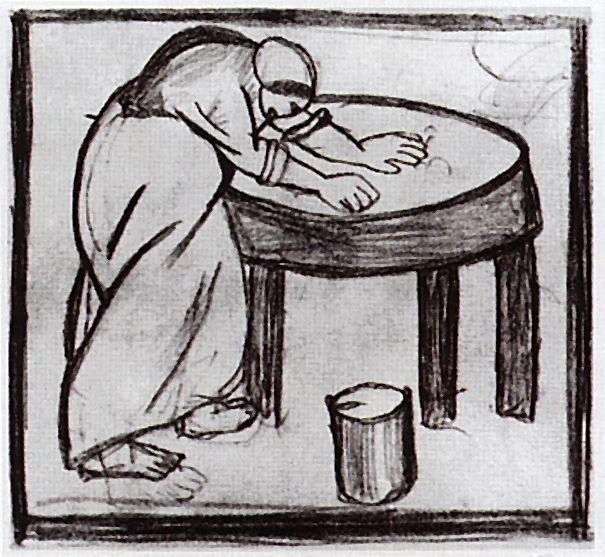This charcoal illustration, with a black-painted border, captures a somewhat distorted, yet evocative scene from what appears to be the late 1700s to early 1800s. Centered within the image is a woman, dressed in a simple, robe-like gown and a bonnet covering her head. Her attire, stretching from her ankles to her forearms, harks back to an old-fashioned, possibly maid-like appearance. The woman is barefoot and her posture is hunched over, suggesting she's engaged in strenuous activity.

She leans over a large, round table, her hands pressing firmly onto its surface as if she's scrubbing it or cleaning something within it. The table, with three visible legs and a notably thick structure, appears almost as tall as she is, further distorting the scene's perspective. Below the table lies a cylindrical bucket or can, perhaps holding the cleaning fluid she’s using, and a log of wood rests beside the table, resembling a stool.

The sketch strikes a balance between simplicity and oddity, presenting an elongated figure in a primitive, perhaps intentionally naive, artistic style. The black-and-white composition, bordered unevenly with thick brushstrokes, reinforces the rustic, aged ambiance of the piece.